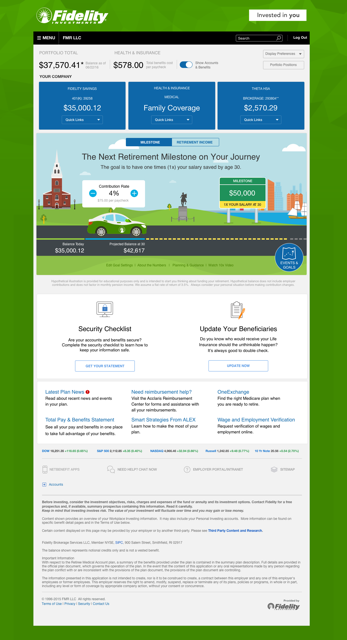This screenshot features a vivid green background with a central large white rectangle. Positioned above the rectangle is a company logo rendered in white, accompanied by "Fidelity" to its right. On the right-hand side of the image, a white box contains the phrase "Invested in You" in black text.

The primary white rectangle begins with a black bar across its top, transitioning into a light gray background as the section progresses downward. This segment includes some text and a toggle switch. Following this, three horizontal blue rectangles appear, each adorned with light blue text.

Beneath the blue rectangles, a computer-generated image depicts a car navigating a road, a church in the background, a street sign, and several buildings. Some black text accompanies this image. Below it, two evenly spaced icons are presented, one on the left and one on the right, each with black text identifying them and a black sentence beneath.

Further down, two rectangular buttons outlined in blue feature light blue text inside. Subsequently, three columns of blue and black text are arranged below. At the very bottom of the screen, fine black writing, reminiscent of the footer text common to website pages, concludes the composition.